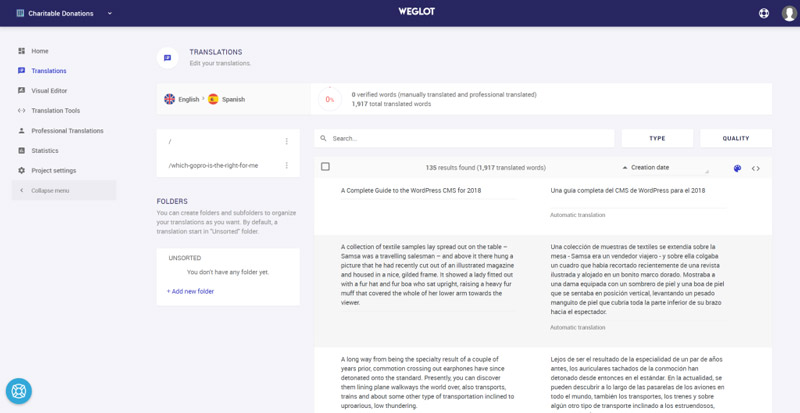This is a detailed screenshot of the website Weglot. At the top of the image is a thin blue bar that stretches across the screen, prominently displaying the site name, "Weglot," in the center.

In the upper left-hand corner of the blue bar, there is a section labeled "Charitable Donations" accompanied by a drop-down arrow. 

The left side of the screenshot features a vertical menu with several options listed: 

1. Home 
2. Translations 
3. Visual Editor 
4. Translation Tools 
5. Professional Translations 
6. Statistics 
7. Project Settings

Additionally, there is a category menu with a back arrow at the top of this vertical menu.

The main content area, located to the right of the vertical menu, is headed with the word "Translations" in the top left corner. Directly underneath this heading, the text reads "Edit your translations." 

Below this text is a white box containing the options for English and Spanish. Each language has a circular symbol next to it, with the Spanish language option being represented by the Spanish flag.

Another white box is situated below the language selection area. Further down, there is a section labeled "Folders."